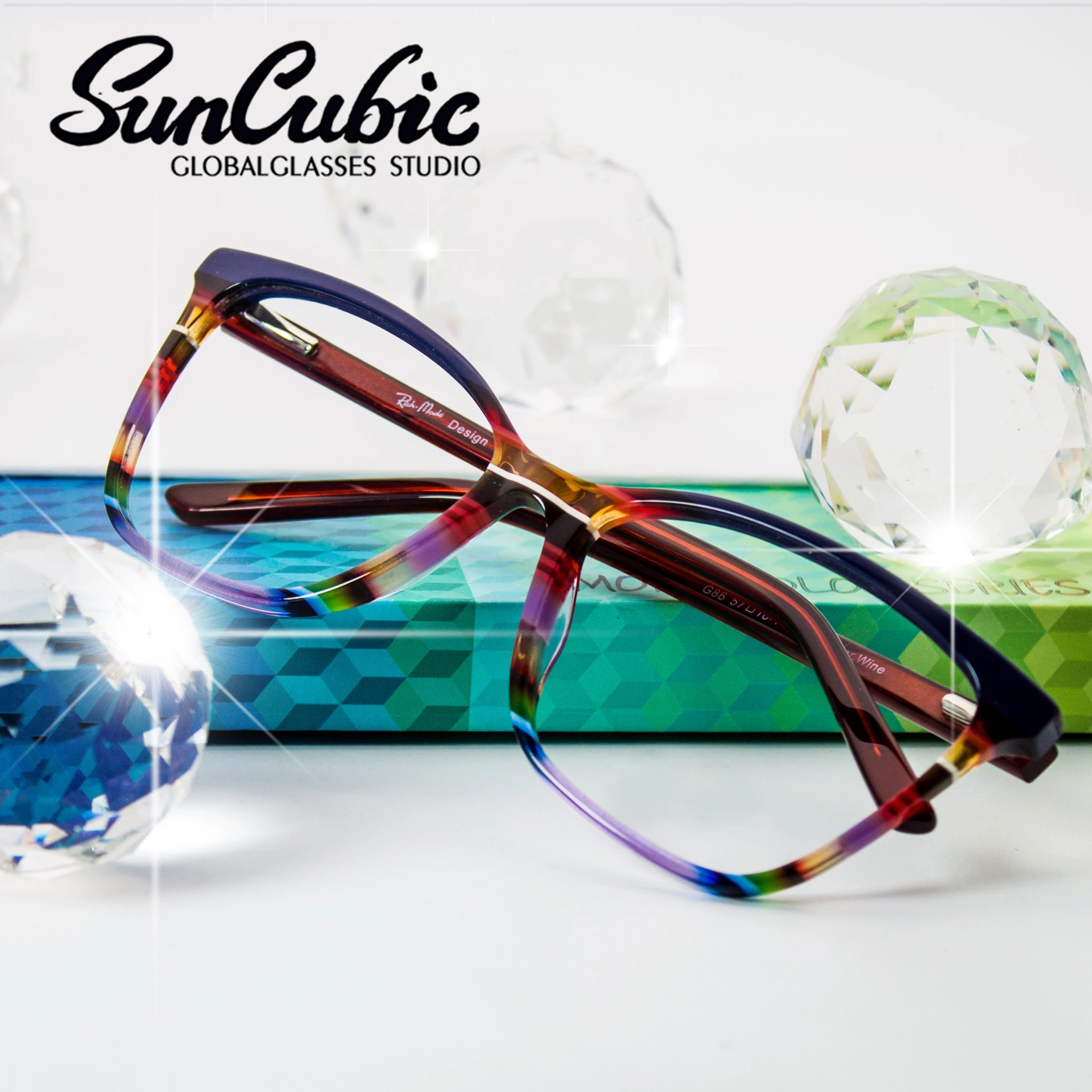This detailed advertisement features a pair of eyeglasses from Sun Cubic Global Glasses Studio. The setting is highly professional, designed to attract attention with its array of vivid and elegant elements. The eyeglass frames are prominently displayed at the center of the image. They showcase a striking multicolored design, starting with blue and transitioning through shades of red, purple, and green. The bridge of the frames is a complex blend of purple, red, black, and white, while the temples, although partially obscured due to their folded position, display a sophisticated brown hue.

One frame rests on the ground, while the other leans against a multicolored blue-green box, possibly the packaging for the glasses. This box features dynamic colors like blue, green, and yellow, enhancing the overall visual appeal. Surrounding the frames are several diamond balls—one notably large diamond ball in the front and several in the background—all reflecting light, adding a touch of luxury and brilliance.

In the upper left corner of the advertisement, the text "Sun Cubic Global Glasses Studio" is displayed in bold black letters, grounding the image in its brand identity. The intricate details and colorful design of the glasses, combined with the elegant backdrop of reflective diamonds, create a captivating and luxurious visual narrative tailored for a high-end audience.